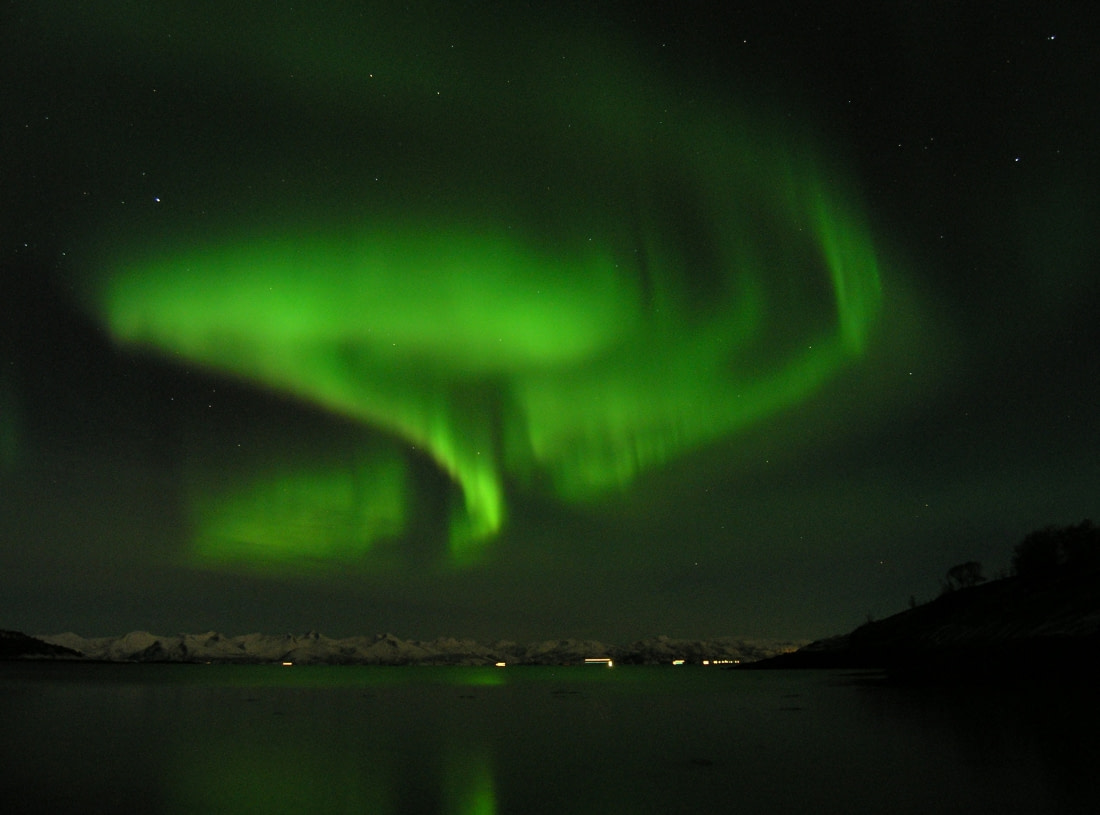In this nighttime photo, the dark sky is alive with the mesmerizing green swirls of the northern lights, creating a vibrant display against a backdrop of twinkling white stars. In the middle of the image, this ethereal green aura accentuates the horizon, casting a luminous glow over the scene. Below the sky, a still body of water reflects the northern lights, giving a sense of symmetry and doubling the enchanting green hue. On the far-right side, there is a gradual upward slope, possibly a hillside, leading out of the frame. At the water's edge, you can discern distant mountains with a faint white-gray appearance, and scattered lights suggestive of houses or artificial sources. The overall setting is tranquil, with the water and sky combining to create a serene yet captivating natural spectacle.